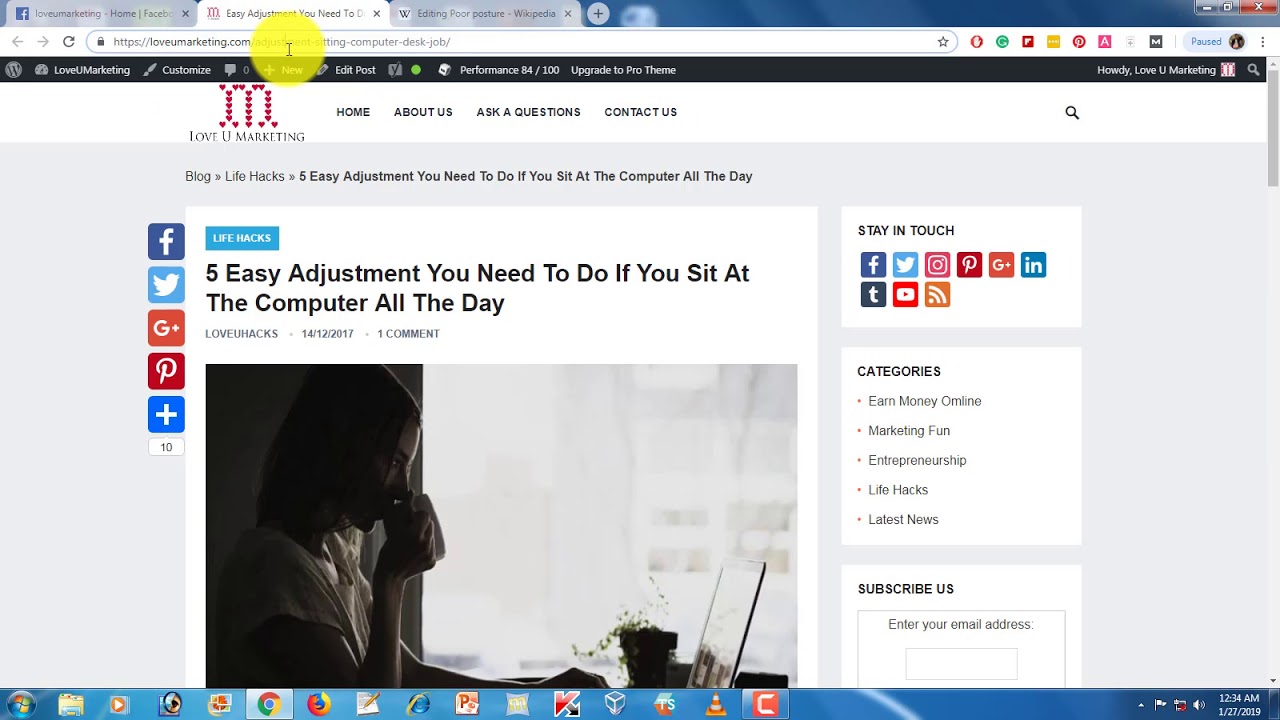This image captures a screenshot of an older version of the Windows operating system, likely Windows 7, as indicated by the legacy Microsoft logo located in the lower-left corner. At the top of the screen, there's a standard menu bar and three open browser tabs. The URL visible in the address bar appears to be from lovejmarketing.com, featuring an article titled "Five Easy Adjustments You Need to Do If You Sit at the Computer All Day," categorized under life hacks. The article provides tips to improve posture and back health for individuals who spend prolonged hours at a computer.

The web page layout includes a sidebar on the left featuring social media icons for Facebook, Twitter, and Google+, allowing readers to share the content. Similarly, on the right side, there are additional options to stay connected through social media. Below this, the website displays various categories, including "Earn Money Online," "Marketing Fun," "Entrepreneurship," "Life Hacks," and "Latest News." There's also a subscription section where users can enter their email address to stay updated.

The taskbar at the bottom of the screen shows approximately ten open windows, including the Chrome browser in use. Additional browser icons for Firefox, Internet Explorer, and others are also present. Overall, the screenshot showcases a typical website browsing experience on an older version of the Windows operating system.